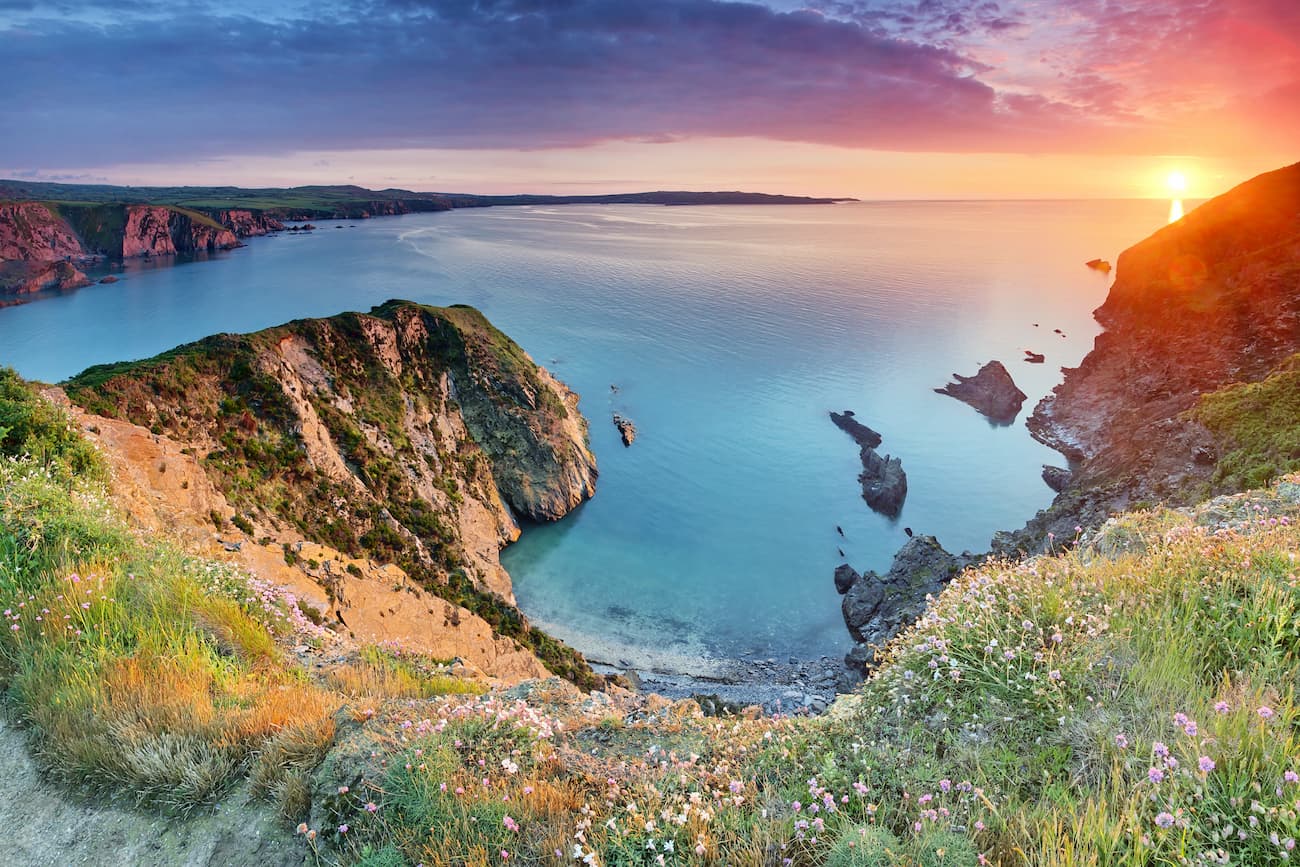A stunning photograph capturing an evening sunset over a bright blue sea. The sky is a mesmerizing blend of blue, purple, pink, red, yellow, and orange hues as the sun sets towards the bottom right corner. Dominating the scene, a large, sandy hillside lined with patches of green grass and small, colorful flowers—ranging from pink to yellow, orange, and purple—descends towards the expansive body of water. To the far left, faint outlines of additional rock-strewn hills create a grayish, shadowy presence, suggesting distant structures partially hidden from view. The water shimmers in a gradient of blue, transitioning to whitish hues where gentle waves break upon the shore. Along the cliff edges are rocky surfaces accented with algae, adding rich texture to the landscape. The image's upper portion reveals darkening clouds as night approaches, completing this picturesque setting with an array of natural beauty and vibrant colors.